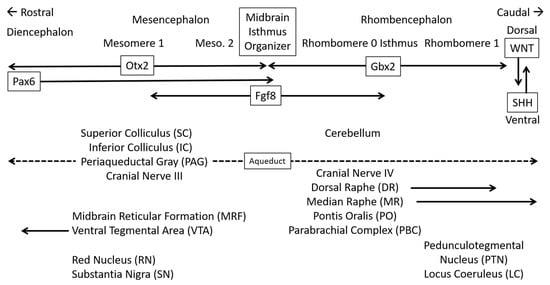The image depicts a highly detailed and complex flow chart or diagram on a white background, filled with blue text and numerous arrows. It appears to detail a biological process, likely related to brain structures and pathways, and is highly specialized, probably intended for advanced students or medical professionals. The main terms include rostral diencephalon, mesomere 1 and 2, mesencephalon, midbrain isthmus organizer, rhombomere 0 and 1, rhombencephalon, isthmus, and caudal regions with directional labels like dorsal and ventral. Key components such as WNT and SHH are highlighted with arrows indicating their interactions. The chart includes critical brain regions and structures like the cerebellum, superior and inferior colliculus, periaqueductal gray, cranial nerves 3 and 4, various raphe nuclei, pontus oralis, parabrachial complex, midbrain reticular formation, ventral tegmental area, red nucleus, substantia nigra, pedunculopontine tegmental nucleus, and locus coeruleus. The layout is intricate, with arrows pointing in various directions, indicating a sophisticated network of biological connections and processes, emblematic of a medical or scientific diagram found in advanced textbooks.